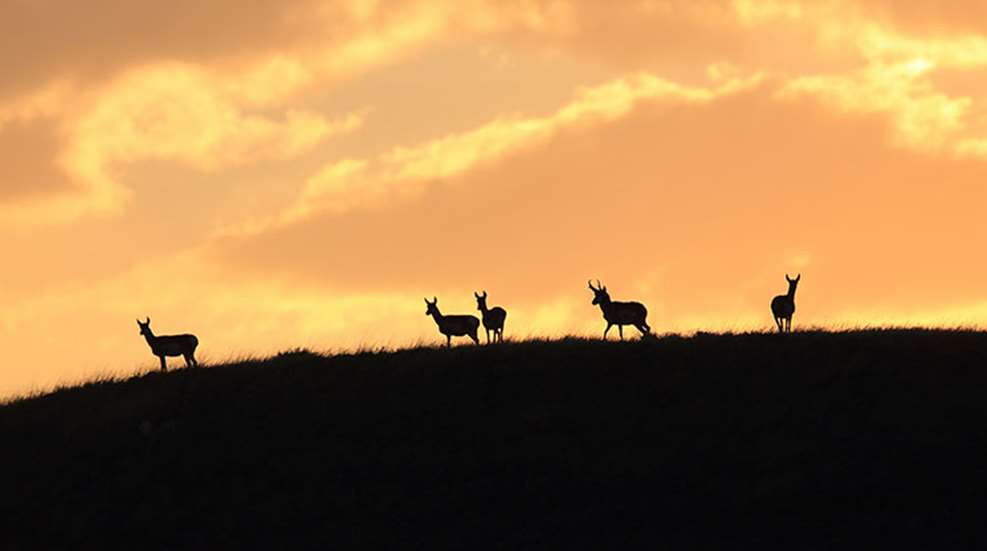In this striking image, five deer are silhouetted against a vivid sunset. The sky is painted in deep and bright oranges, with clouds adding texture and contrast. Four of the deer are does, standing together, while the second from the right is a buck, distinguishable by his antlers. The grassy plain they're standing on is cloaked in darkness, making the deer appear as black silhouettes. The unique lighting creates a breathtaking scene where the only illuminated elements are the intensely colored sky and the edges of the clouds. This composition captures a moment of serene beauty as the day transitions into night.